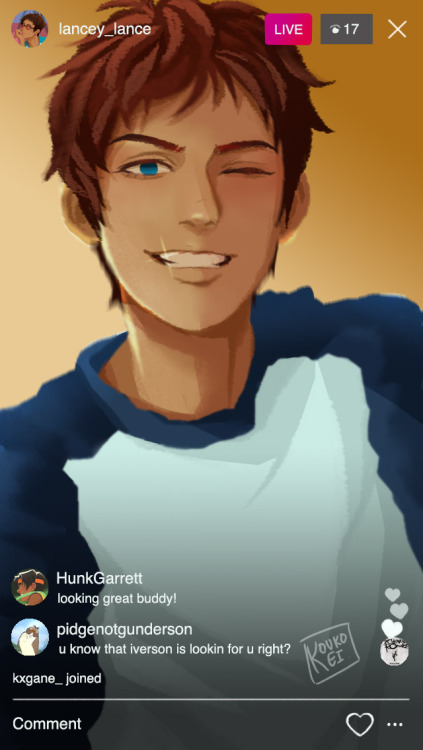Instagram Live Screenshot: A detailed depiction of an Instagram Live session showing the profile of user "lancy_lance" with a cartoon-themed profile picture located in a circular frame in the top left corner. The live broadcast is noted by a "LIVE" button beside the username, and it indicates that 17 people are currently watching. An "X" icon is seen in the top right corner, presumably to exit the live session.

At the center of the image is an AI-generated cartoon of a male figure with short, brown hair, and blue eyes. He is Caucasian, winking with one eye closed and smiling broadly, revealing bright white teeth with a noticeable glint. The background features a tan-brown gradient transitioning from lighter on the left to darker on the right.

Below the main image, ongoing comments from viewers are visible. Highlights include, "Looking great buddy" from user 'hunt_garrett', and "You know Iverson is looking for you right?" from user 'pigeon_not_gunderson'. Additionally, the interface indicates that music by My Chemical Romance (MCR) is playing during this live session.